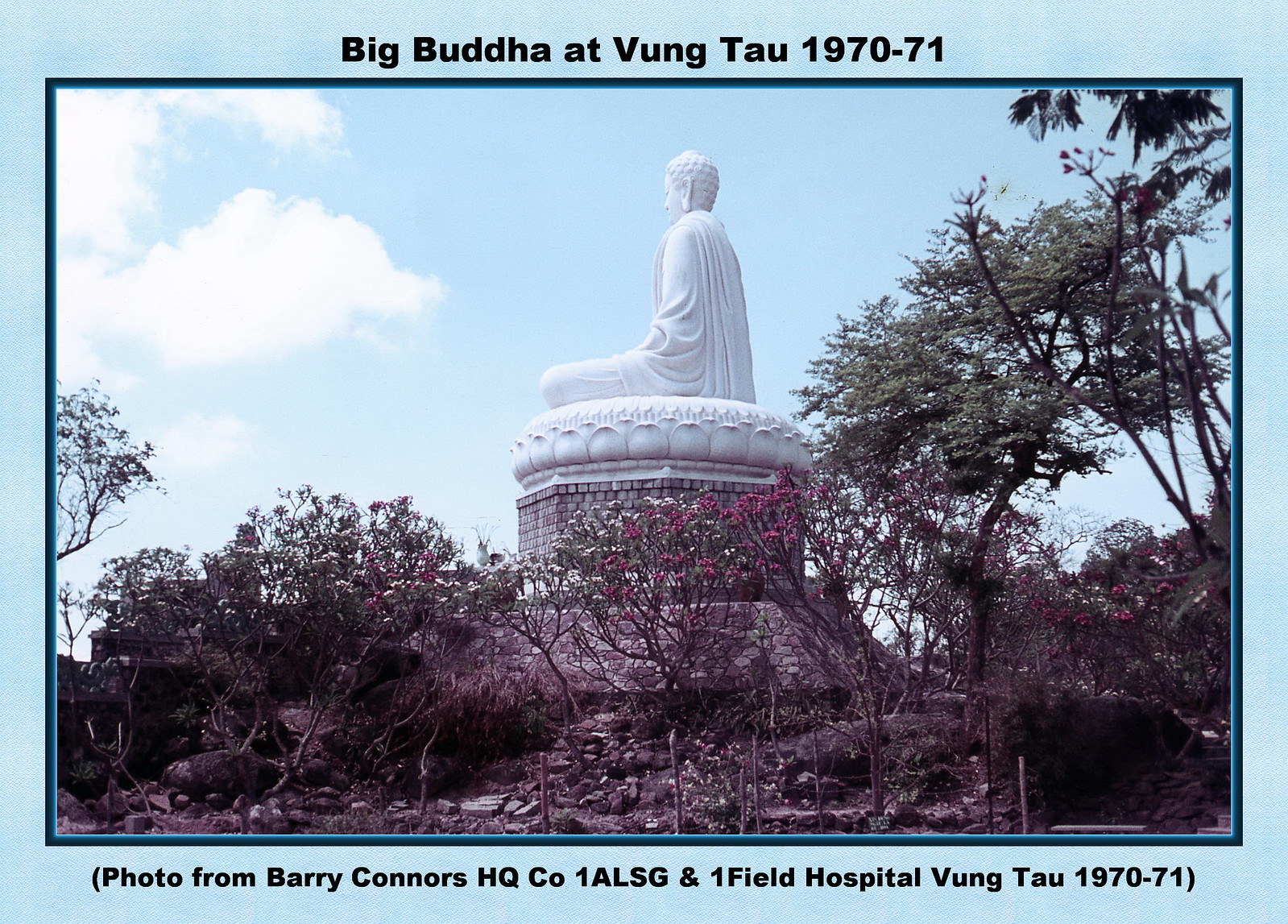This vintage postcard, titled "Big Buddha at Vung Tau 1970-71," showcases a compelling photograph taken by Barry Connors from HQCO 1ALSG and Onefield Hospital Vung Tau in 1970-1971. Encased within a light blue border accented by a darker bold line, the photograph features a side profile of a majestic cement-carved Buddha statue, recognizable by its long ears, curly hair, and flowing robe adorned with a flowery design. The Buddha is seated on a white pedestal which is itself elevated on a circular hexagonal-like brick structure. Surrounding the statue are lush trees adorned with blooming pink and white flowers, set against a backdrop of a pale blue sky adorned with cumulus clouds in the upper left quadrant. The scene vividly captures the serene outdoor setting, devoid of other buildings or people, portraying a tranquil day in Vung Tau during the early 1970s.